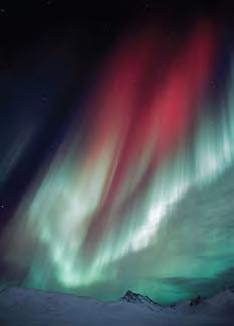This image is a photograph taken at night, showcasing the stunning Aurora Borealis. The photograph, rectangular in shape and measuring about two inches high and one to one and a half inches wide, captures a sky filled with vibrant colors and intricate light formations. At the base of the image, snow-covered mountaintops stretch from the lower left and right corners, rising a quarter of an inch. Above the mountains, streams of light illuminate the sky, predominantly in tones of green that seem to outline additional, partially obscured peaks.

From the center right-hand side of the image, a bright, whitish-green lightning bolt-like light shoots downward toward the mountains before curling back up, interspersed with various green striations. In the center of the image, striking red lights form two large beams, converging and creating an elongated, heart-like shape. The upper part of the sky is dominated by deep black tones, interspersed with hints of blue and purple, particularly along the left side and blending towards the heart-shaped red lights. The overall effect is a mesmerizing mix of green, red, blue, and purple hues, painting the night sky in vivid, otherworldly colors.